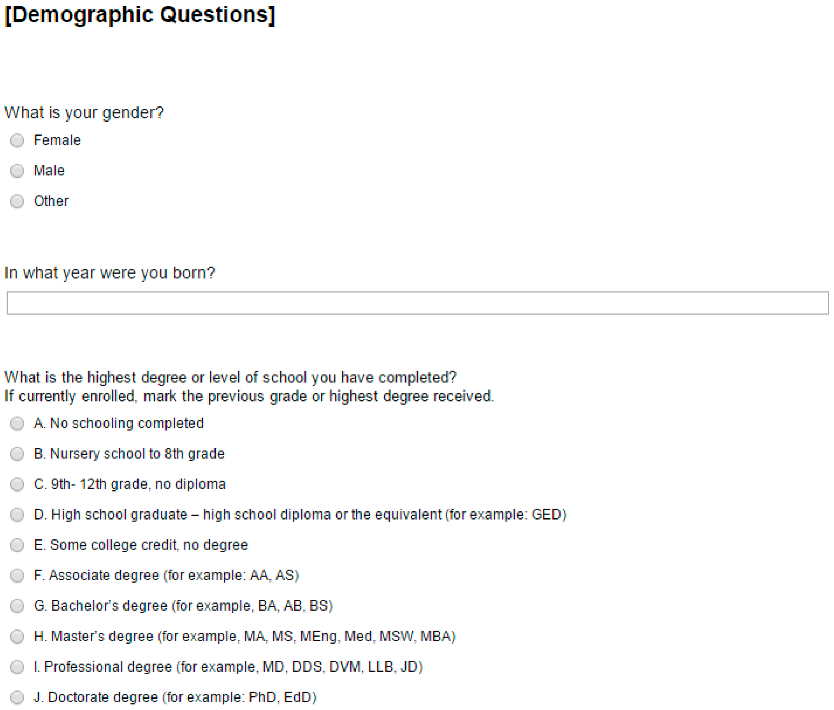A detailed caption for the image could be:

"The screenshot displays a demographic questionnaire section. At the top in bold black text, it reads 'Demographic Questions.' Directly below, smaller and slightly less bold black text poses the query, 'What is your gender?' followed by three options: Female, Male, and Other, each accompanied by a radio button. The next question asks, 'In what year were you born?' with an open rectangular text field spanning the full width of the screen for the response. Below that, another question reads, 'What is the highest degree or level of school you have completed? If currently enrolled, mark the previous grade or highest degree received.' This section offers options labeled from A to J, each with corresponding radio buttons. Option A is 'No schooling completed,' Option B is 'Nursery school to 5th grade,' Option C is '9th to 12th grade, no diploma,' Option D is 'High school graduate, high school diploma or the equivalent (e.g., GED),' Option E is 'Some college credit, no degree,' Option F is 'Associate degree (e.g., AA, AS),' Option G is 'Bachelor’s degree (e.g., BA, AB, BS),' Option H is 'Master’s degree (e.g., MA, MS, MEng, MEd, MSW, MBA),' Option I is 'Professional degree (e.g., MD, DDS, DVM, LLB, JD),' and Option J is 'Doctorate degree (e.g., PhD, EdD).' Each option is clearly marked with a radio button to the left."